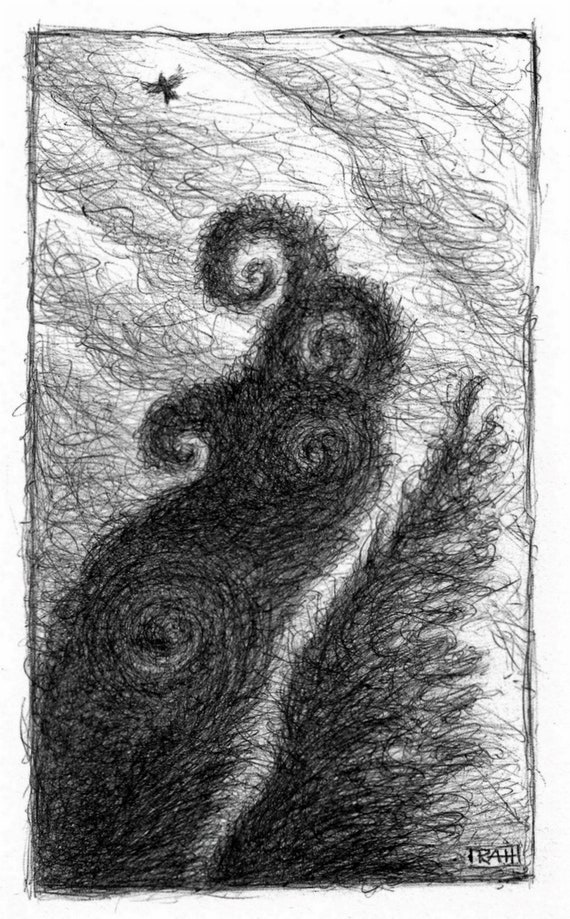The intricate image is a scratch pen drawing on a white sheet of paper, predominantly black and white with varying intensities of black strokes. It features a small bird at the top left corner, potentially a shadow or silhouette, drawn in a delicate and barely-there manner. The main focal point is an enormous, eldritch-like monster resembling a dragon or a giant, crocodile-like creature. The monster's large, gaping mouth extends from the top to off the page, adorned with spiraling nostrils and a dark swirl where its eye might be. The overall composition suggests swirling, chaotic energy, possibly evoking a sense of high winds or movement akin to an ocean's treacherous waves or trees thrashing in a storm. The rough, etched black border frames the piece, and the artist's signature is placed at the bottom right, grounding the surreal and dynamic imagery.